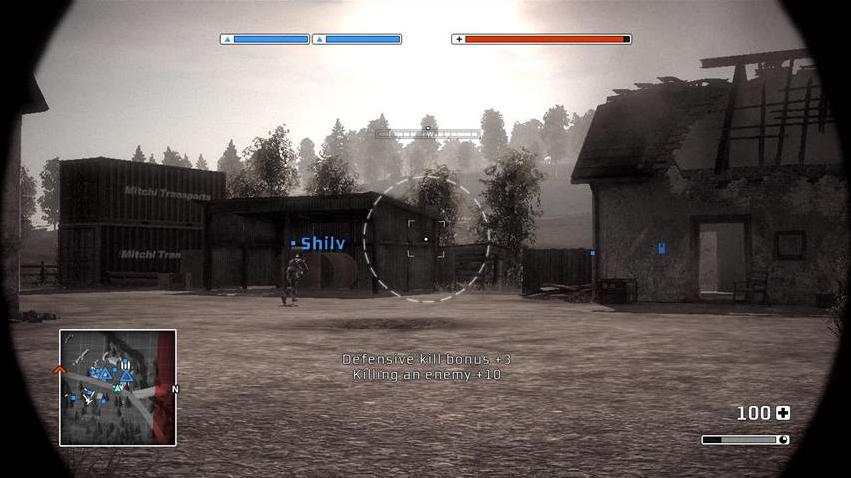This image appears to be a screenshot from a first-person shooter video game set in a dilapidated outdoor environment. The scene depicts the player navigating through an abandoned industrial area that shows signs of severe damage from a past fire, with large sections of the roof missing. Two large storage containers and an open-air barn with multiple holes in its roof can be seen in the background.

In the user interface at the top of the screen, there are three meters: one red meter, mostly filled with a small section missing, and two fully filled blue meters positioned adjacent to each other. These likely represent the player's health and shield status. Next to a character figure, the word "SHIELD" is displayed in blue text.

The player is aiming through a firearm's sight, which features a reticle to assist with accurate targeting. A map located at the bottom of the screen provides navigational assistance, marked with various indicators to help complete objectives. The HUD (Heads-Up Display) also shows gameplay statistics and bonuses, including a notification reading "DEF KILL BONUS +3, KILLING AN ENEMY +10."